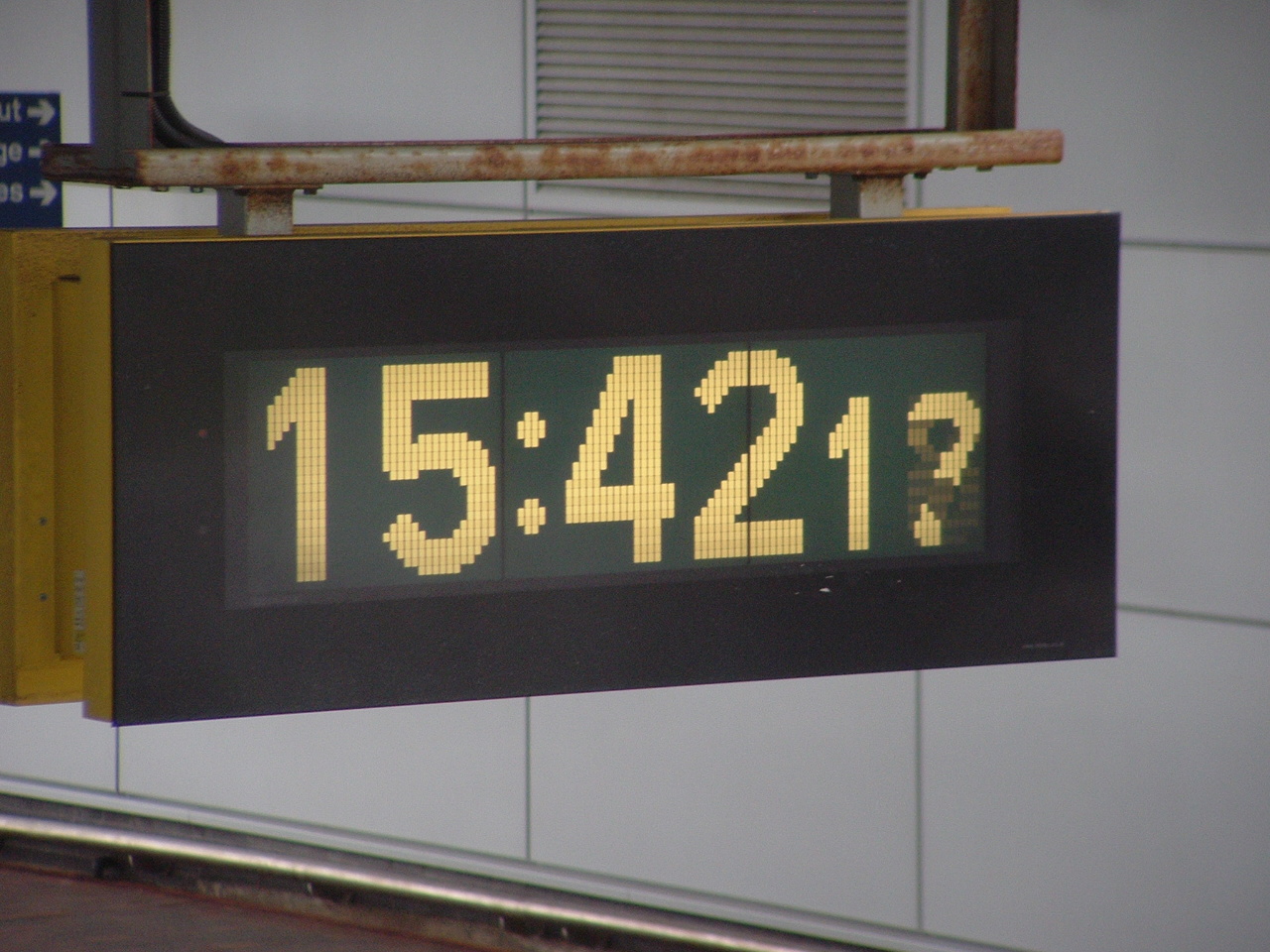This vibrant color photograph is taken outdoors, capturing a large digital street sign. The sign is suspended by a rusty metal sign post extending from its top edge. The back of the digital sign is painted yellow, while its front features a black outline framing illuminated yellow numbers. The digital display shows the numbers "15," "42," and "1," alongside a clock symbol and a partially broken number to the right of the "1."

In the background, a blue sign with white text and directional arrows contrasts against a white building. The positioning and style of the signage suggest it may belong to a bustling city, capturing the juxtaposition of modern digital elements with weather-worn infrastructure.